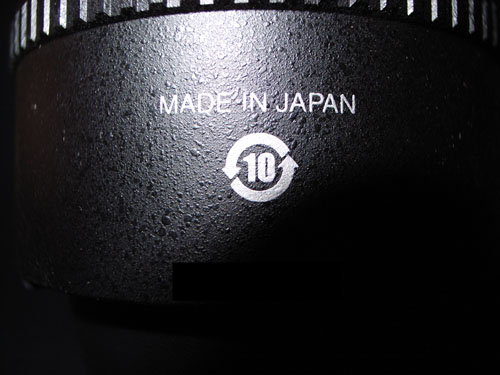This is a highly detailed black-and-white photograph of an unknown cylindrical object, taken at an extremely close range. The object appears to be made of a black metal or possibly a textured plastic composite. Prominently featured in the photograph are the bold, block-printed white words "MADE IN JAPAN," accompanied by a recycling symbol comprising two arrows in a circular formation with the number 10 in the middle.

The cylindrical shape of the object is evident from its curvature, with what looks like "sweaty" wetness or condensation visible on its surface. Gray elements and shadow-like black dots can be seen, adding to the textured appearance. At the top of the cylinder, part of a bolt or component resembling machine gears is visible, with teeth-like structures highlighted by the light source. This light appears to be coming from above and slightly behind the photographer, creating a distinct flair of white and casting shadows.

To the right side and bottom right of the photograph, there is a noticeable shadow, darkening parts of the frame and adding depth to the image. The composition and details give a mysterious and industrial feel, strongly emphasizing the object's man-made origin.